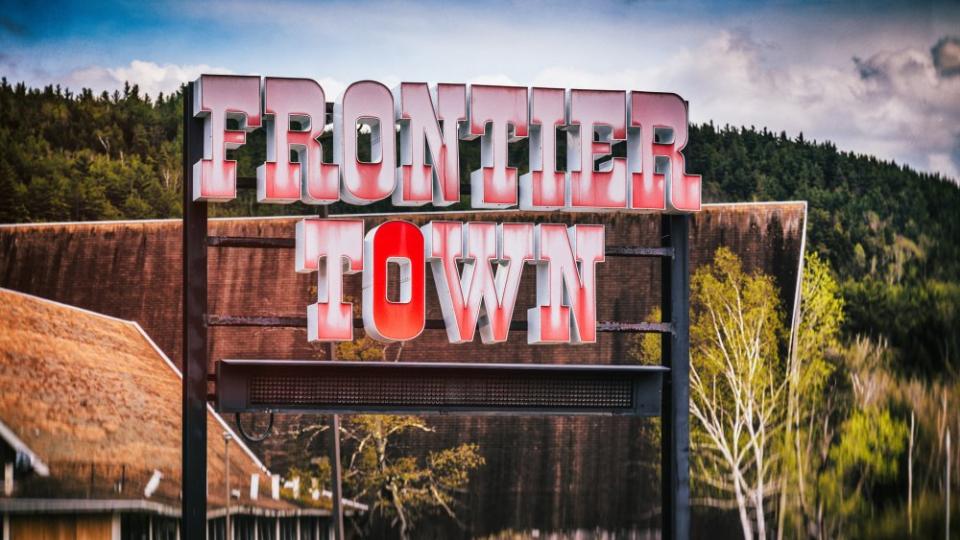This photograph captures a nostalgic scene of a dated signboard standing in front of a series of buildings nestled in a heavily wooded area, set against tree-covered hills. The focal point of the image is a black metal sign, prominently featuring the words "Frontier Town" in once-vibrant red lettering. Over time, most of the red paint has faded to white, leaving only the "O" in "Town" retaining its bright red hue. The buildings in the background are mostly obscured, showing only their tall, arched roofs amidst the dense trees. The sky is heavily clouded, further enveloping the setting in an overcast ambiance.